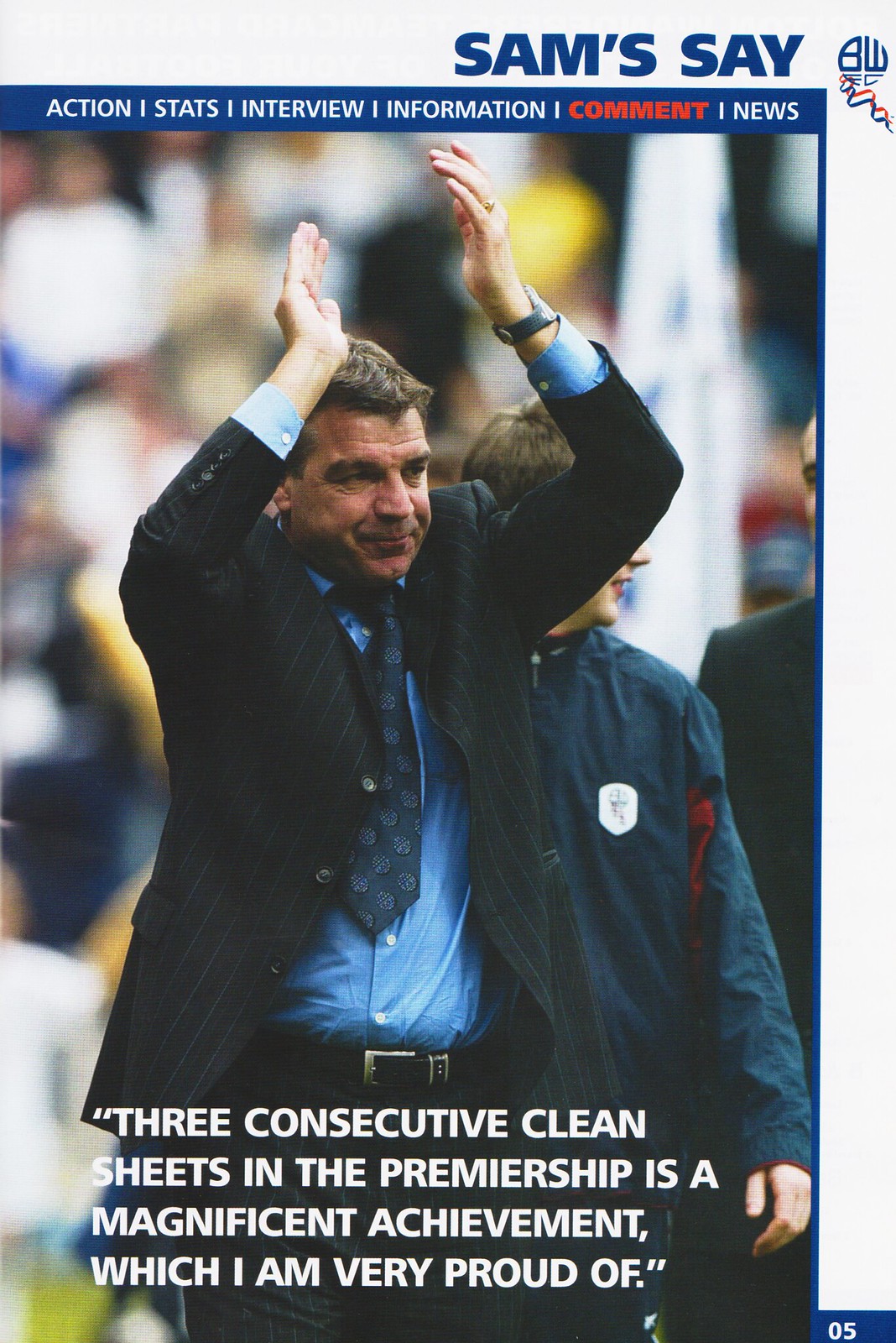The image appears to be an advertisement or a magazine page featuring a middle-aged, Caucasian male coach, presumably of a football (soccer) team, celebrating an achievement. The man, dressed in a nice suit and tie with a blue shirt, is holding his hands above his head as if clapping, possibly acknowledging a significant milestone. Behind him, an out-of-focus crowd can be seen, along with a person in a blue windbreaker. The upper part of the image has a white border with blue text that reads "Sam Say," followed by sections labeled "Action, Stats, Interview, Information, Comment, News." At the bottom of the photo, a quote in white text highlights the coach's pride in achieving "three consecutive clean sheets in the Premiership," which he describes as "a magnificent achievement." In the bottom right corner, a small blue rectangle contains the number "05" in white.